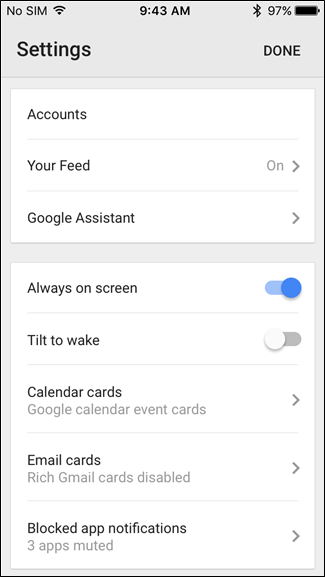This is a detailed photo of the settings page on a cell phone, captured in portrait orientation, making the image much taller than it is wide. The background primarily features shades of gray with several white rectangular elements arranged within it.

At the top of the screen, positioned against a gray backdrop, there is a status bar. On the left side, the text "No SIM" is displayed in black font next to a fully visible black Wi-Fi signal icon. Centrally placed at the top is the current time shown as "9:43 AM". To the right, an icon depicting Bluetooth status is displayed along with a battery indicator at "97%" capacity, where the battery icon is horizontal with a black fill almost reaching full.

Below the status bar, a section separated by a thin gray border shows the word "Settings" in large, bold, black letters on the left, with a "Done" button to the right.

Following this header, the lighter gray background transitions into the main settings menu. The first section displays a white text bubble arranged horizontally with three options in black font, each separated by thin gray lines: "Account," "Your Feed" (which is selected as "On"), and "Google Assistant."

Below this, another white text bubble appears in a portrait orientation, listing additional settings options: "Always On Screen," "Tilt to Wake," "Calendar Cards," "Email Cards," and "Blocks App Notifications." Notably, the "Always On Screen" option has a blue toggle switch set to the right, indicating it is turned on.